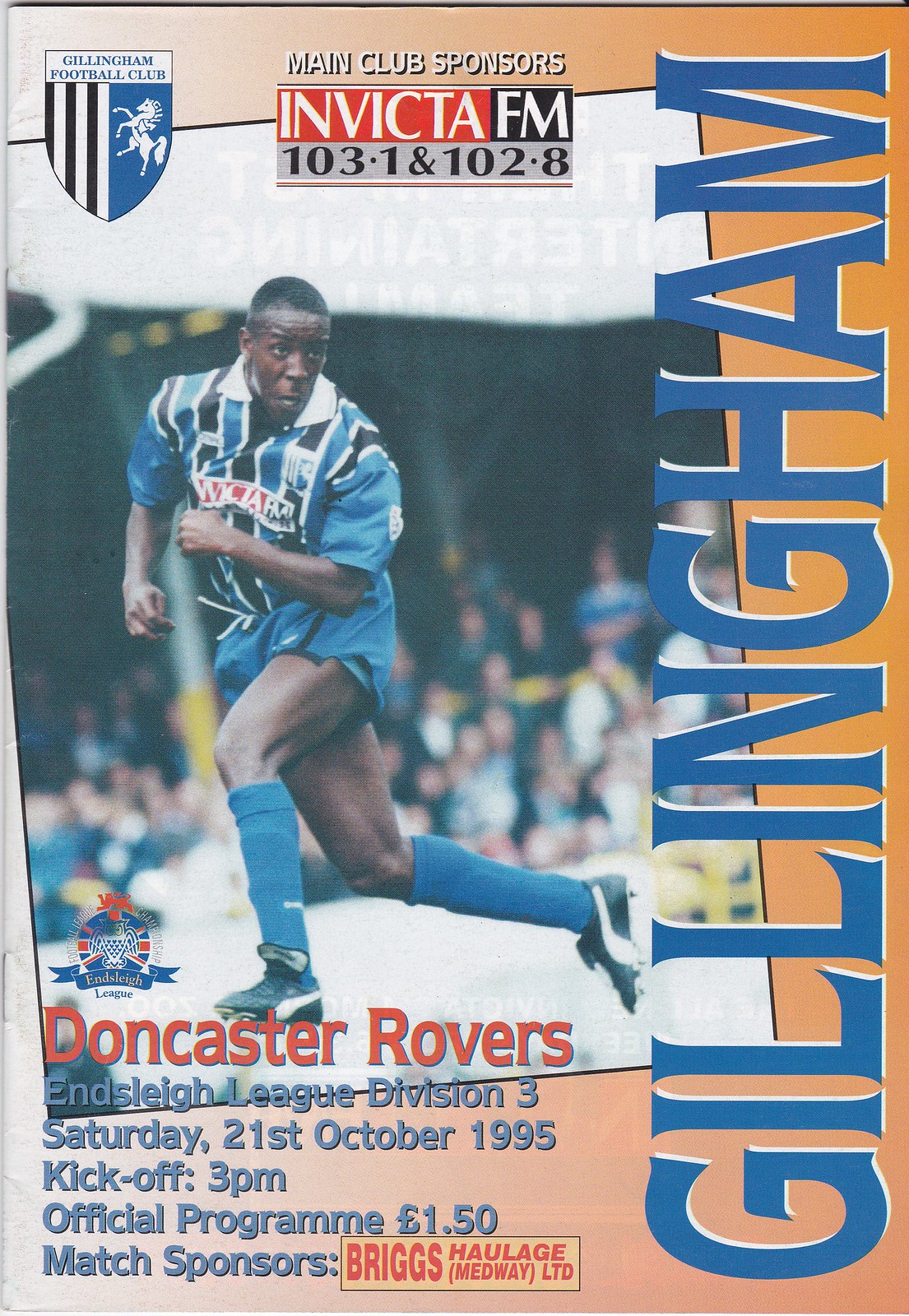This is an image of a soccer program cover featuring a predominantly orange and white background. At the top, it prominently displays the main club sponsors: "Invicta FM 103.1 and 102.8." To the top left, the Gillingham Football Club shield is presented, which features black and white stripes on the left half, and a white horse on a blue background on the right half. The shield is accompanied by the text "Gillingham Football Club."

The central part of the cover showcases a football player in blue, captured in mid-run heading to the left while glancing to the right. Behind the player, the image features an out-of-focus stadium crowd.

At the very bottom, the notation "Doncaster Rovers" appears in red, followed by blue text that reads "Ensley League Division 3, Saturday 21st October 1995, kickoff 3 p.m." Additionally, the official program cost is listed as "£1.50," with match sponsors indicated as "Briggs Haulage Medway Limited." Along the right side of the cover, blue vertical text spells out "Gillingham" from bottom to top.